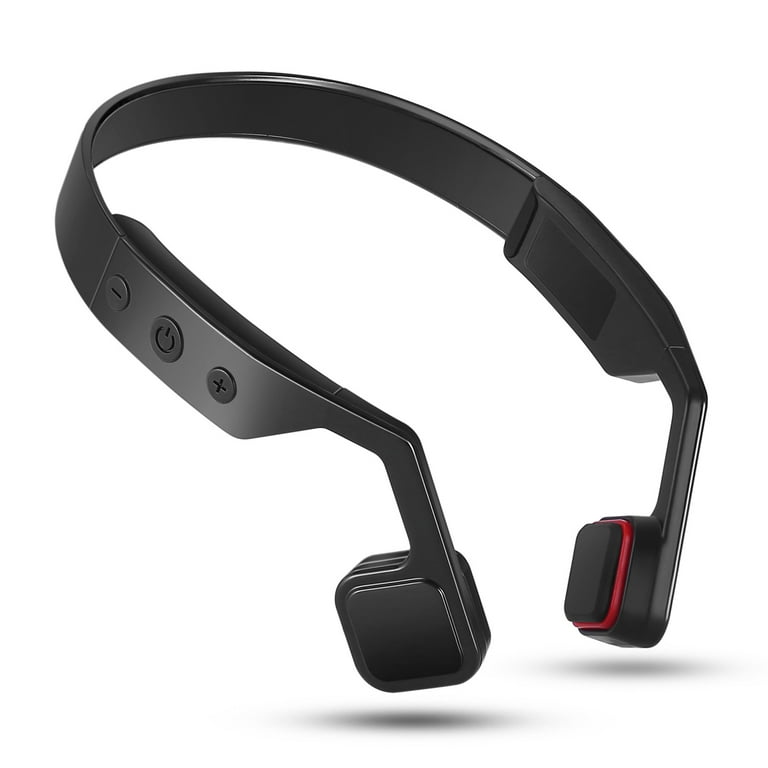This image appears to be an advertisement for a unique pair of Bluetooth headphones. The design is quite unconventional, featuring small, square earpieces instead of the typical round or oval shapes. These earpieces have a distinct red trim around them, adding a pop of color to the otherwise entirely black set. The headband, which also doubles as a neckband, is constructed from a shiny material that might be either plastic or metal, designed with added cushioning to ensure comfort and avoid chafing.

The earpieces potentially function through bone conduction, resting on the jawbone rather than inside the ear canal, which could offer a different listening experience. The headphones feature three circular buttons on the thicker portion of the headband situated above the earpieces—two for volume control (plus and minus) and a central power button. This area likely houses the essential circuitry, given its slightly bulkier build. Overall, the design merges innovative auditory technology with ergonomic considerations, making it a standout product.